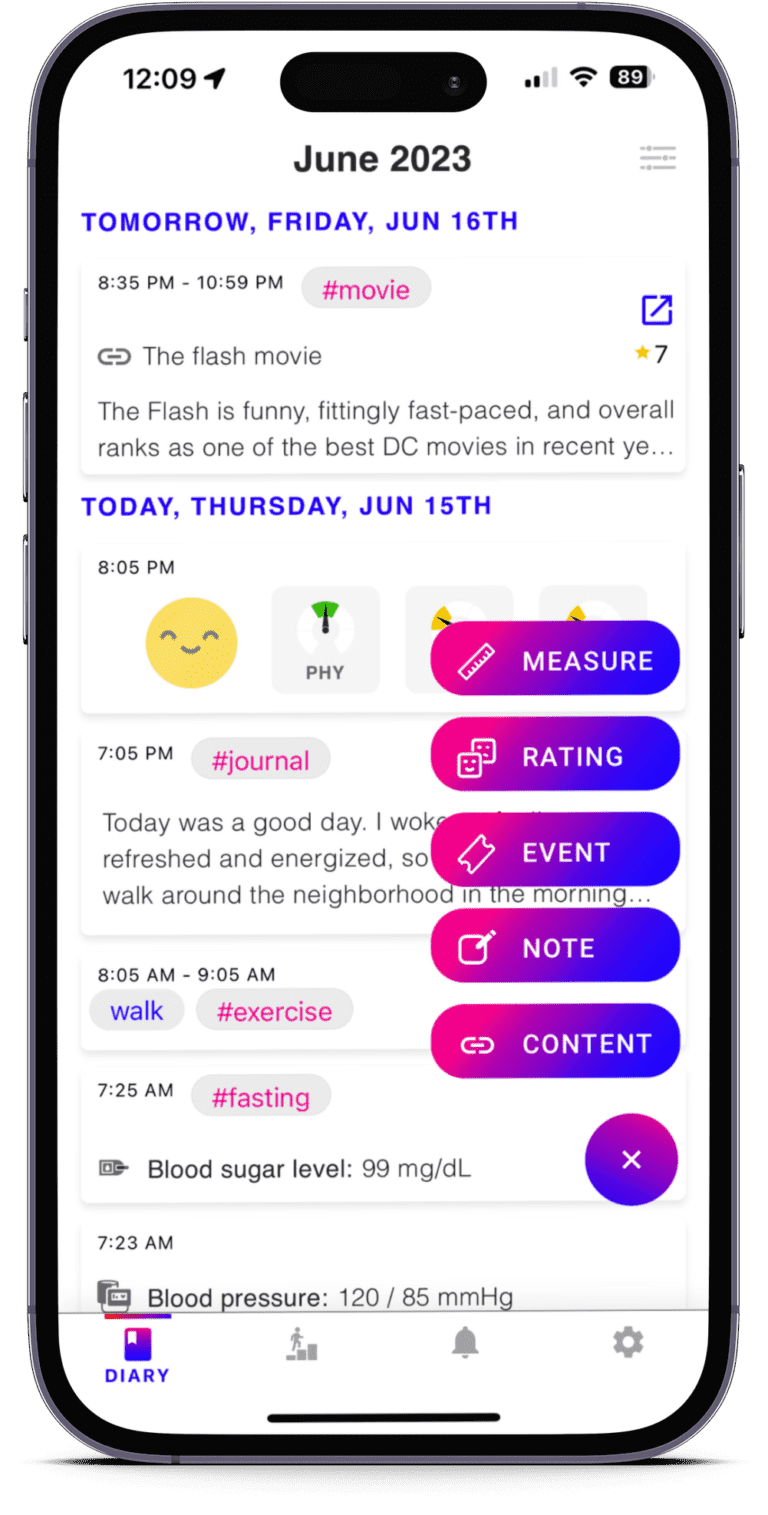A detailed screenshot of a mobile app interface is displayed, likely a calendar or event reminder. At the very top left corner, the current time is indicated as 12:09. To the right, the status bar displays various indicators: two filled bars representing signal strength, a fully filled Wi-Fi icon, and a battery icon showing a charge level of 89%.

Centrally located at the top of the screen, the date is prominently displayed as June 2023. Beneath it, specific event details are provided: "Tomorrow, Friday, June 16th, 8:35 PM to 10:59 PM, #movie, The Flash movie." A brief description reads, "The Flash is funny, fittingly fast-paced, and overall ranks as one of the best DC movies in recent..." However, the description is cut off, leaving the sentence incomplete. 

Just below this event, an entry for "Today, Thursday, June 15th" is visible, though further details are obscured and not fully legible.